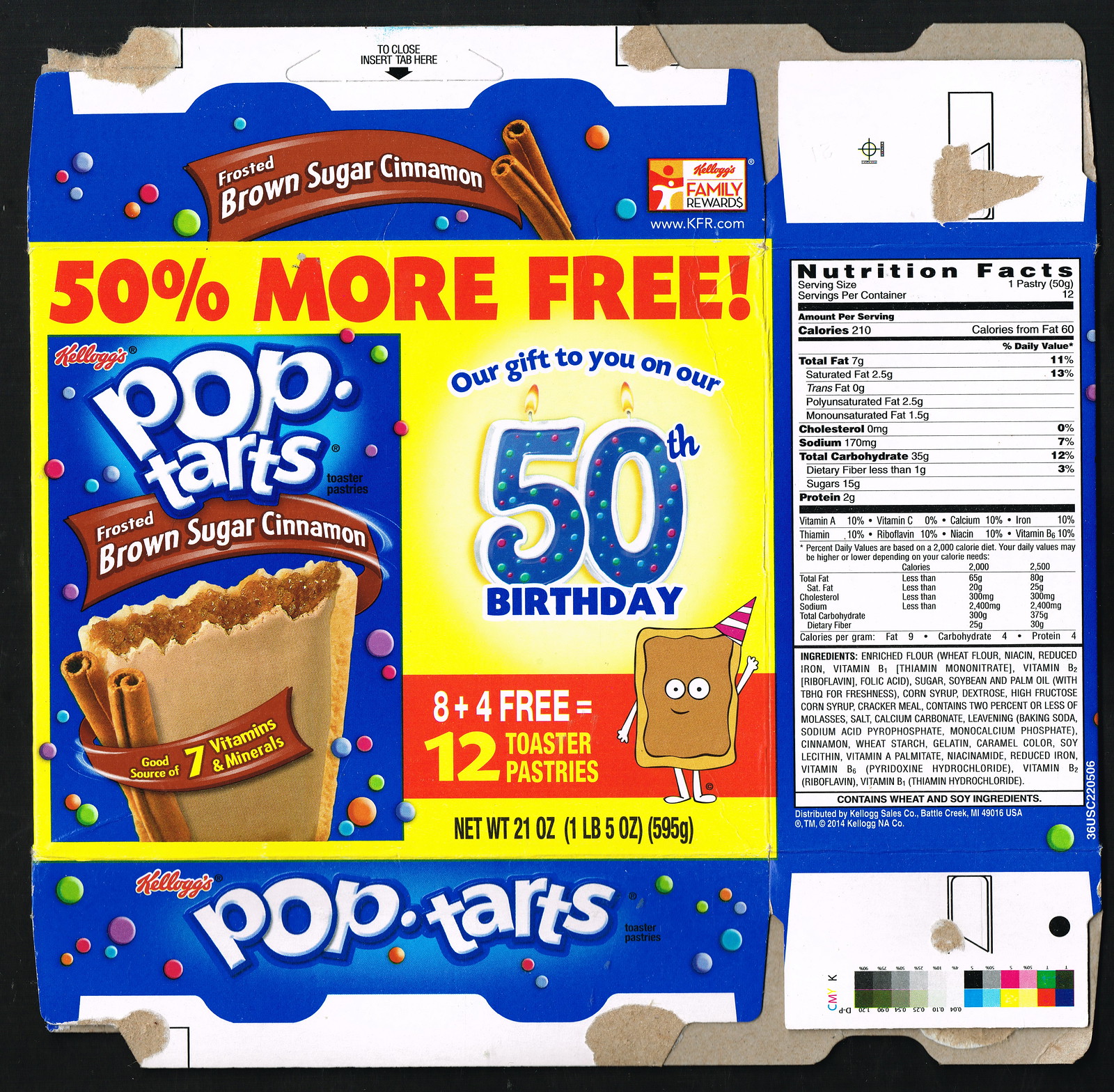This photograph showcases a meticulously flattened Pop-Tart box, specifically of the Frosted Brown Sugar Cinnamon variety. The box has been opened at both ends, revealing glue marks and tear lines where it was originally sealed. At the top of the box, there are graphics featuring two cinnamon sticks and a representation of brown sugar, accompanied by the text "Frosted Brown Sugar Cinnamon" and an advertisement for Kellogg's Family Rewards.

Prominently displayed in the center is a bold statement in red font against a yellow background that reads "50% More Free," celebrating Pop-Tarts' 50th birthday with the message "Our gift to you." A vivid illustration of a Pop-Tart mascot, complete with cheerful eyes, a smile, and a birthday hat, enhances the festive theme. Below this, a broken Pop-Tart showcasing its cinnamon filling underscores the flavor, while the offer, "8 + 4 Free = 12 Toaster Pastries," is highlighted in red and yellow text.

The bottom section of the box reiterates the "Kellogg's Pop-Tarts" branding, with net weight details specified as "21 ounces, 1 pound 5 ounces." On the right-hand side, the nutritional facts are clearly laid out, detailing fat, calories, and other nutritional information. Overall, the flattened box captures an intricate balance of marketing messages, product details, and celebratory elements.